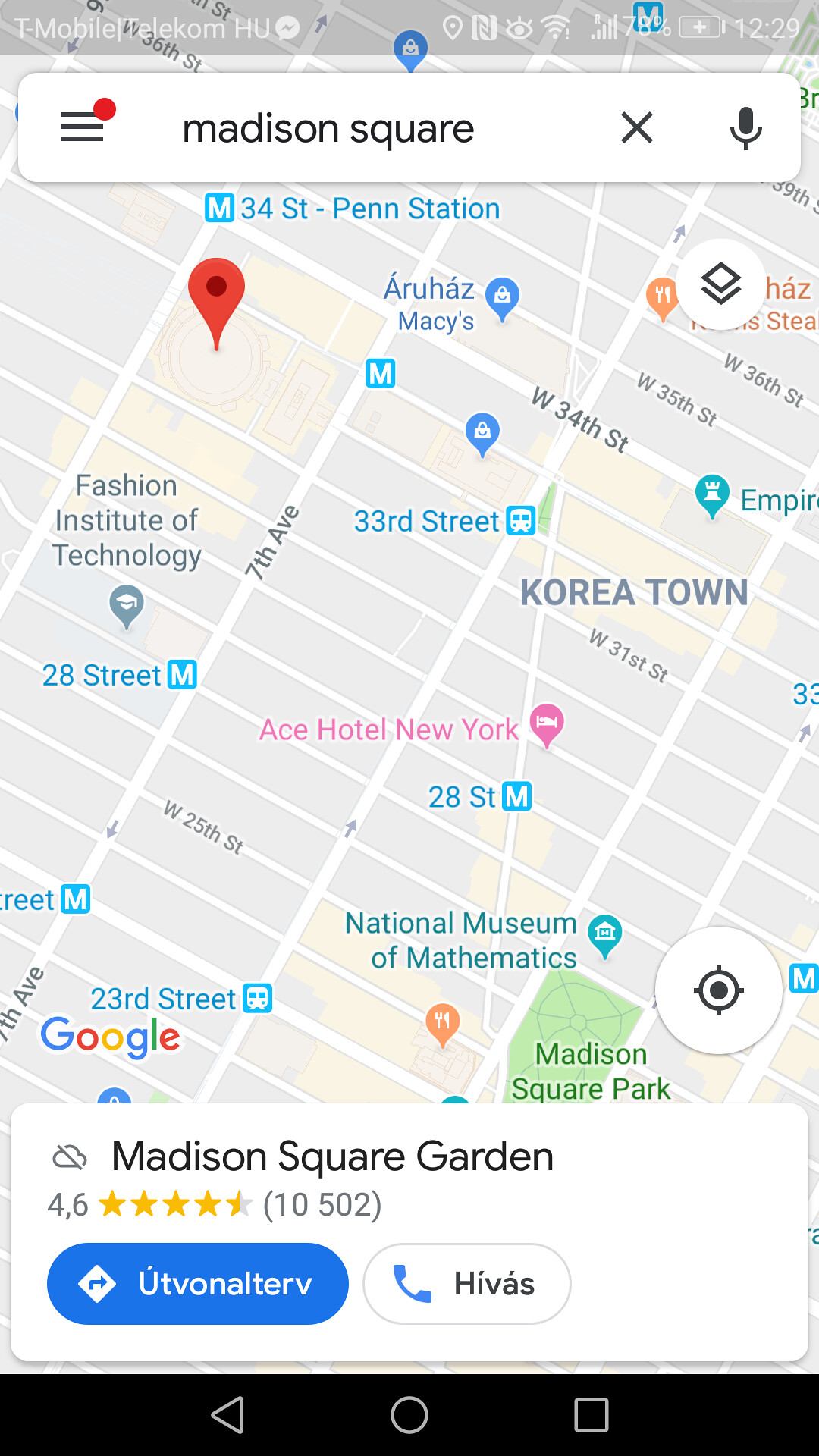The image is a detailed screenshot of a map displayed on a smartphone. At the top of the map, there's a white triangle, and to the left, there's a menu icon with three horizontal lines, accompanied by a small red dot in the upper corner. The title "Madison Square of North Youth Letters" is prominently displayed. 

To the right, there's an "X" icon and next to it, a microphone icon. The main map area showcases a network of streets, some of which are broader and run diagonally from left to right. Directly beneath the title "Madison Square," "34 ST-Penn Station" is labeled, and a red marker is located below this text. To the left of the red marker, the area is predominantly gray, while to the right, a location marked "R. Ross Macy's" is indicated. Adjacent to it on the right side is an icon featuring a white circle, a black square within the circle, and a black triangle below it.

Further down, the word "Koreatown" is written in large letters. Below Koreatown, "Ace Hotel New York" is highlighted in pink, paired with a nearby place marker. At the very bottom of the map, a yellow rectangle labels "Madison Square Garden." To the left of this label, a cloud icon with an arrow through it is visible, accompanied by the numbers "4, 6."

A rating system appears below, with four solid yellow stars and one half-yellow star, followed by the numbers "(10-5-0-2)". Beneath the rating, there is a blue button and a white button, both featuring text in a foreign language; the white button also has a phone icon on it.

At the very bottom of the image, a black navigation bar is present. This bar contains an arrow pointing left, a circle in the middle, and a square icon.

This detailed map screenshot seems to be highlighting various notable locations and features, catering to someone possibly navigating or exploring the Madison Square area.